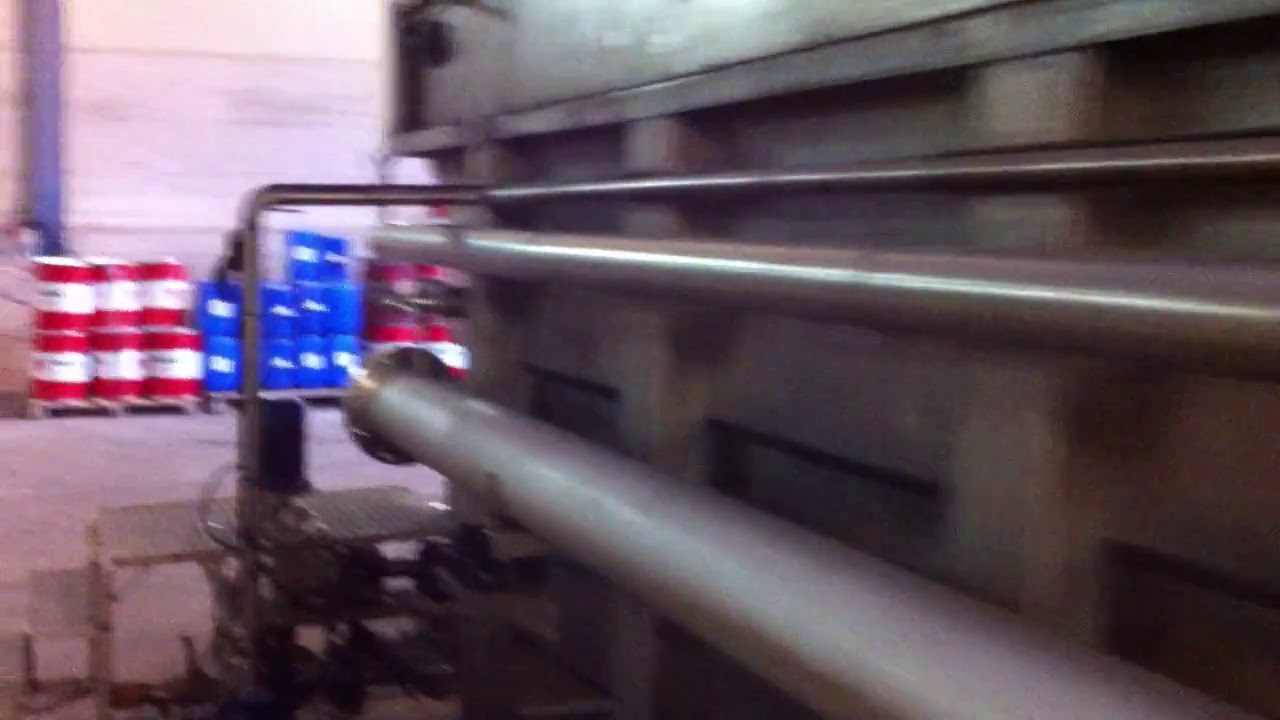The blurry photograph depicts an industrial warehouse or factory scene with several large metal pipes prominently stretching from the bottom right corner towards the center. The pipes, made of silver metal, include two large pipes at the bottom and a smaller, thinner one on top. These pipes are positioned against a gray wall or piece of machinery, accompanying additional pipes extending outward.

The setting features a graded metal platform in front of the pipes, equipped with a railing bar at the top. The ground beneath is a plain, gray cement floor. To the left of the pipes, one can observe machinery parts.

In the background, large canisters are stacked against a beige wall, forming two stacks of red and white canisters and three stacks of blue ones. Also, there are wooden pallets on the floor holding blue metal drums and white metal drums with red stripes on the top and bottom. The image hints at a far-off, blurry window behind these elements, contributing to the overall impression of a complex, cluttered industrial environment.